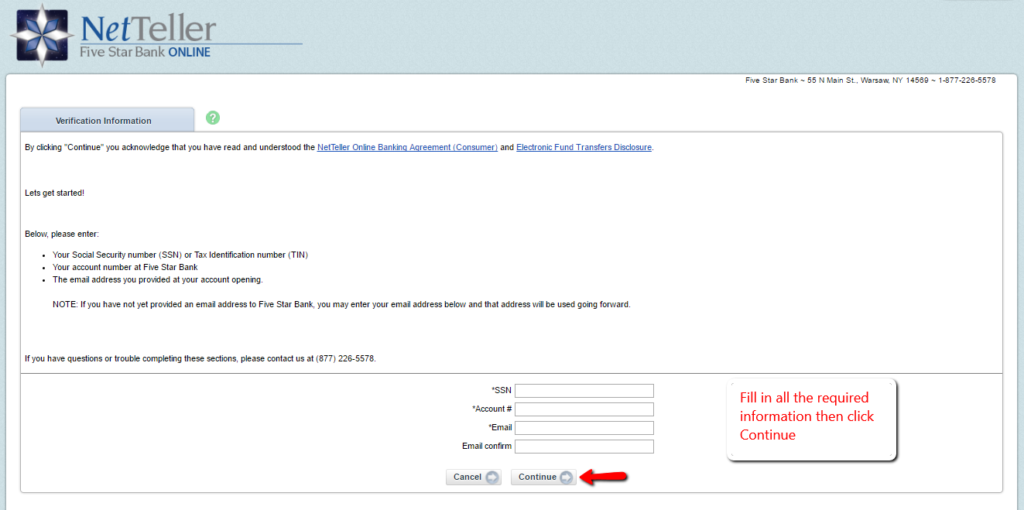Screenshot of a web page from Neteller, showcasing a clean design with a white background. A pastel blue horizontal bar spans the top, featuring a white and blue flower icon set against a black square on the left side. Adjacent to the icon, the word "Neteller" is displayed in blue and gray, with the tagline "Five Star Bank Online" beneath it. 

The main body of the page continues with a white background, where a sidebar tab on the left stands out with its pale blue color. This tab is labeled "Verification Information" and includes a small white question mark inside a green circle, providing additional information. Beneath this, a text section informs users that by clicking "Continue," they acknowledge reading and understanding the Neteller Online Banking Agreements, including Consumer and Electronic Fund Transfer disclosures.